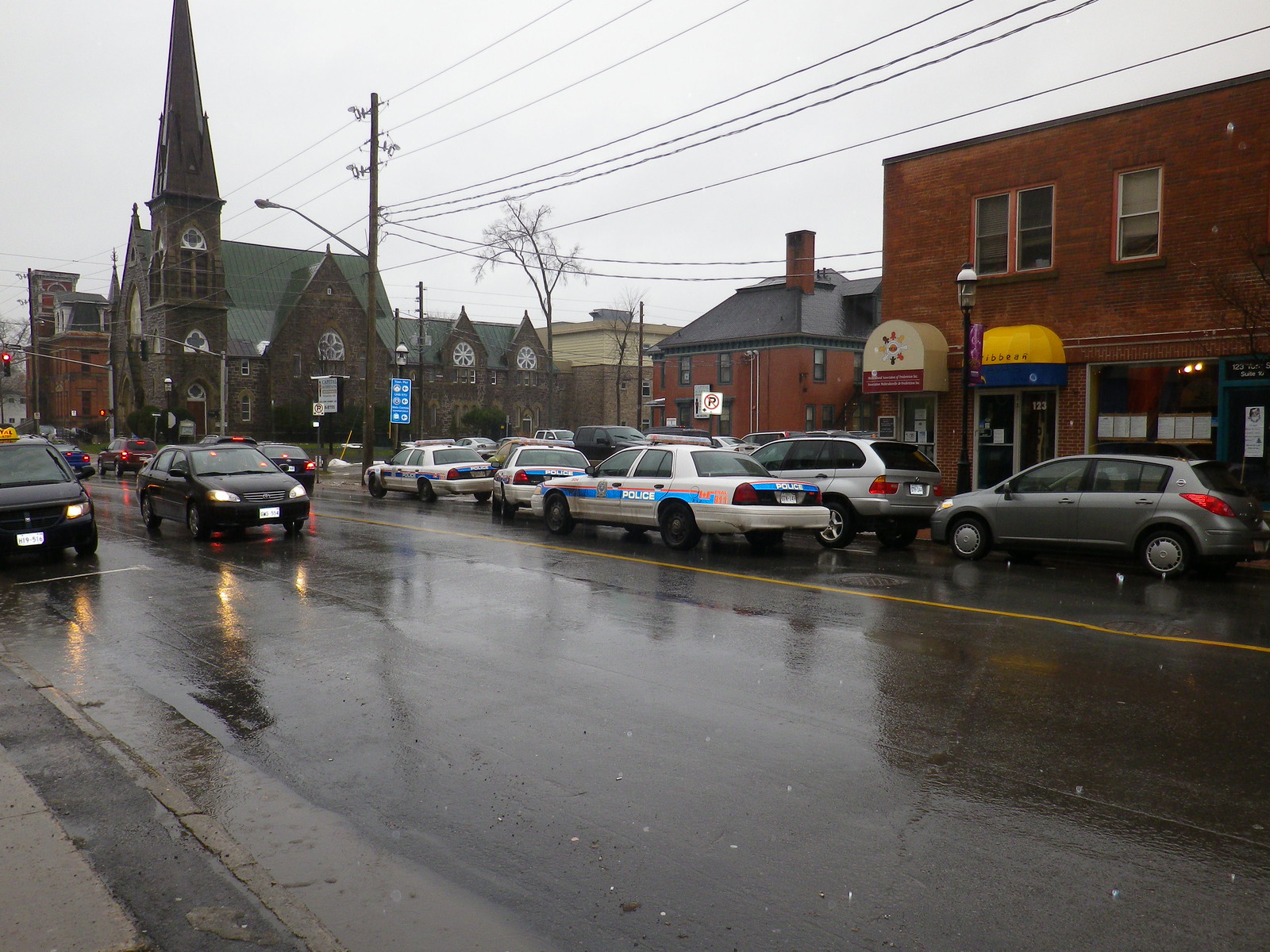The photograph depicts a rainy day on a city street, possibly in Boston. The wet streets reflect the array of vehicles, adding a mirror-like effect to the scene. In the foreground, two black vehicles with their headlights on move towards the viewer. A dividing yellow line splits the lane, with several cars, including three distinctive 80s-style Boston police cruisers, traveling in the opposite direction. These police cars, identified by their white paint and light blue striping with the word "POLICE," are a central feature of the image. To the left side, taillights create a red trail in the wet street. 

Dominating the backdrop is an old brick church with a tall steeple made of dark brown natural stone, reaching high into the light gray sky filled with rain clouds. Surrounding the church, additional red brick buildings contribute to the city's architectural texture. To the far right, a building with a protruding tan awning with colorful designs, and just beside it, another building with a dark blue base and an orangey-yellow top, add a burst of color to the otherwise muted palette of the scene. Overhead, phone lines and a street lamp complete this intricate depiction of an urban street captured amidst a downpour.